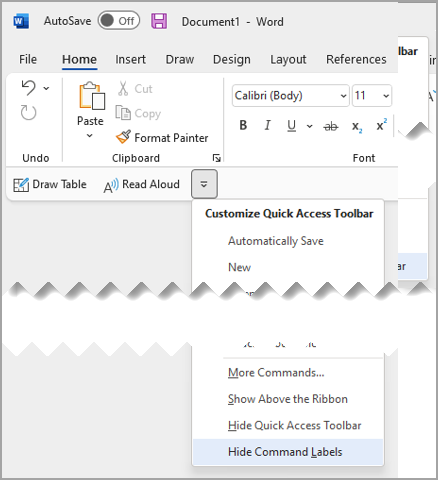This image is a cropped screenshot of a Microsoft Word interface, showcasing the top-left section of the screen. The top-left corner features the familiar Word logo, a white "W" against a blue background, followed by the "AutoSave" option, which is toggled off. Next to it sits a pink floppy disk icon and the text "Document 1 - Word."

Directly below, a gray bar displays a series of menu options in black text: "File," "Home" (which is underlined, indicating it is currently selected), "Insert," "Draw," "Design," "Layout," "References," and more. Underneath this bar, within the white workspace area, several commands and tools are visible. These include options for "Undo," "Paste," "Format Painter," "Clipboard," "Copy," and "Cut." On the right side, font settings are displayed, including "Calibri" font, size 11, and buttons for bold, italics, and underline.

Further down, two arrows point towards a white rectangle housing additional black-text options like "Customize Quick Access Toolbar," "Automatically Save," "New," "More Commands," "Show Above the Ribbon," "Hide Quick Access Toolbar," and "Hide Command Labels."

The image has a notable zigzag pattern at the bottom, suggesting it has been cropped or edited, giving a somewhat fragmented appearance as if from two combined screenshots.